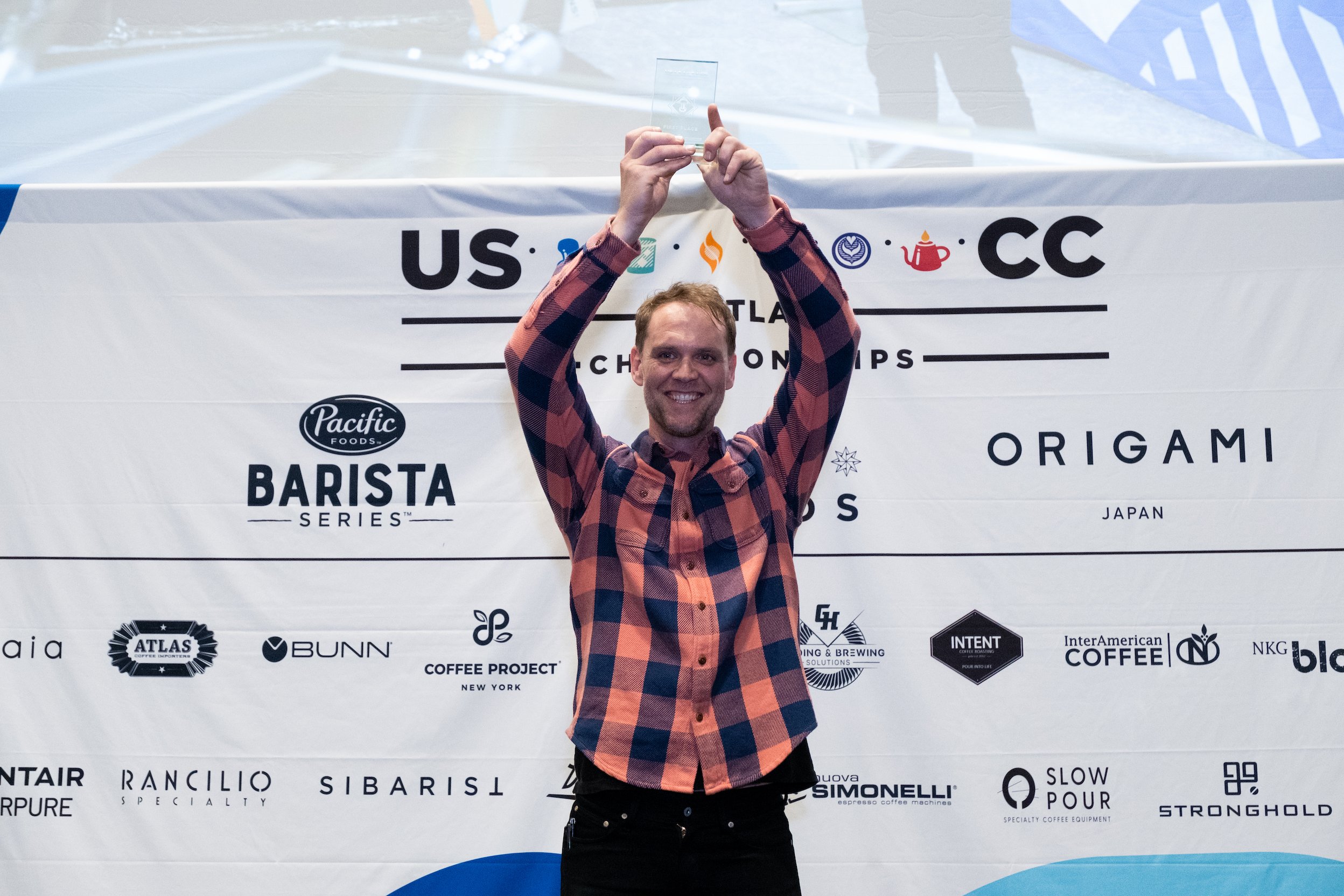In this image, a happy Caucasian man with blonde hair and a goatee stands triumphantly in front of a large white banner filled with numerous advertisements and sponsor logos. He is wearing a red, pinkish-red, and blue flannel shirt paired with black pants. The man is smiling broadly and holding a clear glass trophy high above his head, celebrating what appears to be a significant win. The banner behind him features predominantly black lettering and includes brand names such as Pacific Foods, Barista Series, Origami Japan, Atlas, Bun, Coffee Project, Inter-American Coffee, Intent, Simonelli, Slowpour, Stronghold, and others, suggesting a sponsored event or competition. The banner also mentions "U.S." and "CC", likely part of the event's name, which could be related to championships, given the celebratory context. This detailed scene captures the joyous moment of victory against a backdrop of sponsors and supporters.